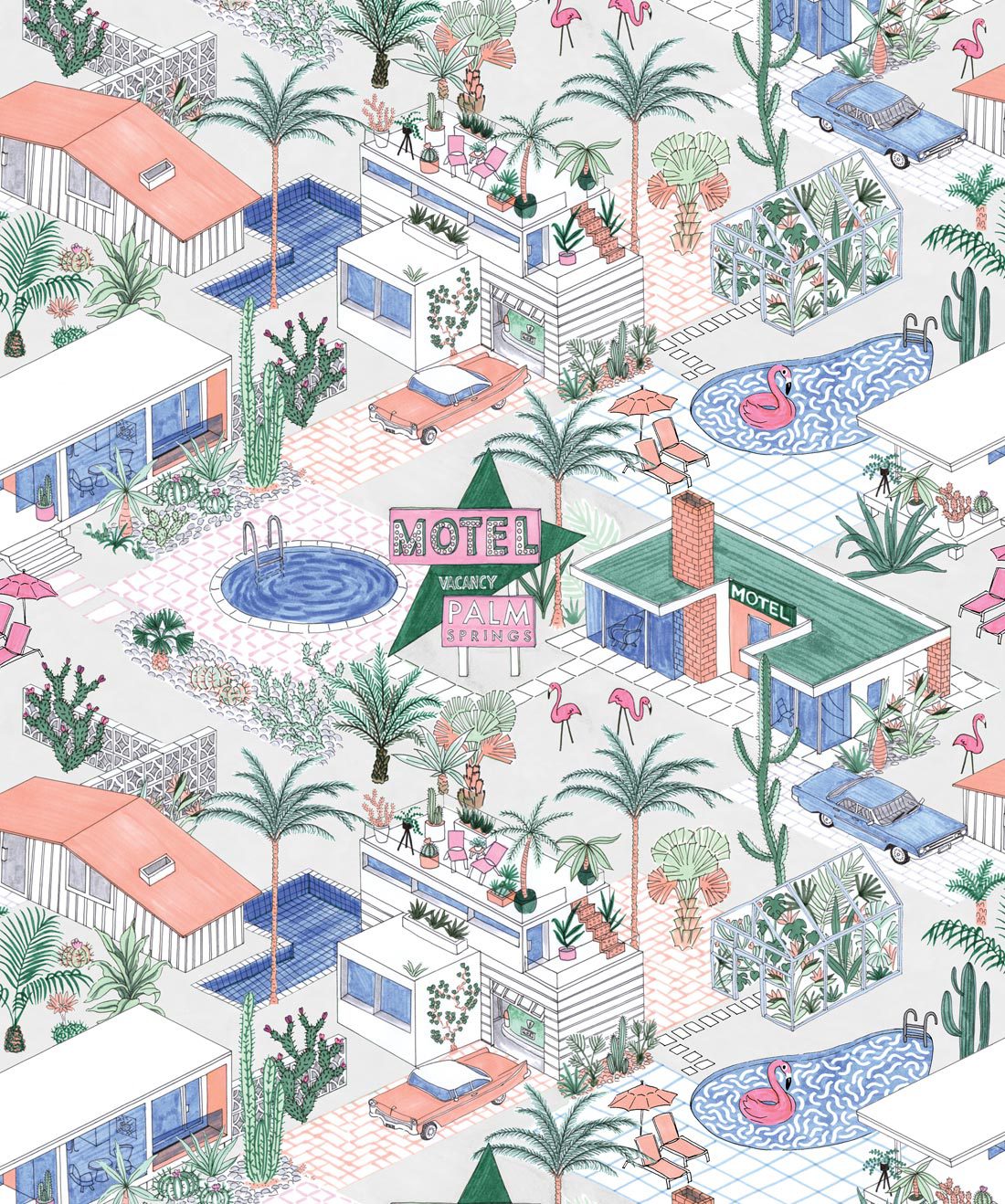This intricately detailed pen and ink illustration showcases a whimsical, map-like layout of a mid-century modern Palm Springs town, rendered in a minimalistic color palette of white, gray, blue, green, and coral. Captured from a three-quarter overhead view, the scene is reminiscent of a town map in a video game, featuring a variety of buildings and elements repeated in a pattern that might adorn fabric. Central to the image is a sign reading "Motel Vacancy, Palm Springs," surrounded by U-shaped motels with green roofs and accompanying kidney-shaped pools with pink flamingo floats.

The illustration includes mid-century houses with distinct details: a white house with an orange roof and small skylight, a rectangular white house with large windows and steps, and a garage with an old-time orange car. The landscape is lush with palm trees, cactuses, and more pink flamingos, enhancing the tropical theme. Pools are meticulously depicted—circular, kidney-shaped, and L-shaped—adding to the town's vibrant character. The use of limited colors brings cohesion and a unique charm to the overall depiction, making it both visually striking and nostalgically quaint.